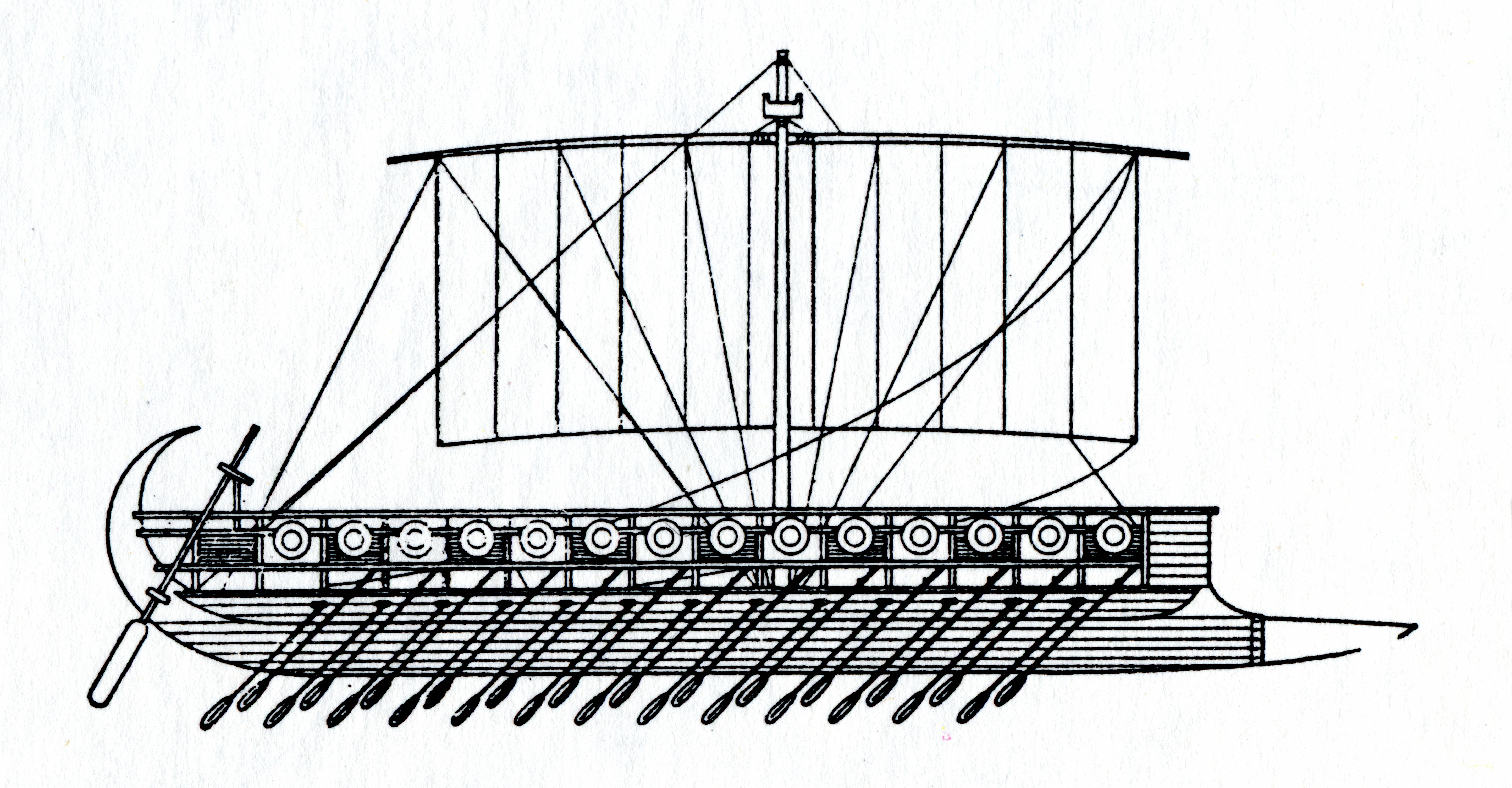The image features a black and white side view illustration of a Viking-style ship, set against a light blue, off-white background with no borders. The rectangular image, approximately five to six inches wide and three inches high, showcases the ship centrally, measuring about three-quarters of an inch in height. The bow of the ship curls upward into a crescent moon shape on the left, while the stern on the right has a large oar, serving as a rudder for steering.

Along the top of the ship, there are small circular details that resemble portholes or possibly cannons. Below these are numerous black oars, extending downward, with a total of 28 oars—14 on each side—indicating where the crew would row to propel the vessel. 

Dominating the center of the ship is a mast, standing a little over an inch tall, with a crossbeam that spans about two inches wide. A large rectangular sail hangs below the crossbeam, completing the ship's navigation apparatus. The detailed illustration predominantly uses black ink on a white background to emphasize its elements, with significant contrasts highlighting the vessel's features.